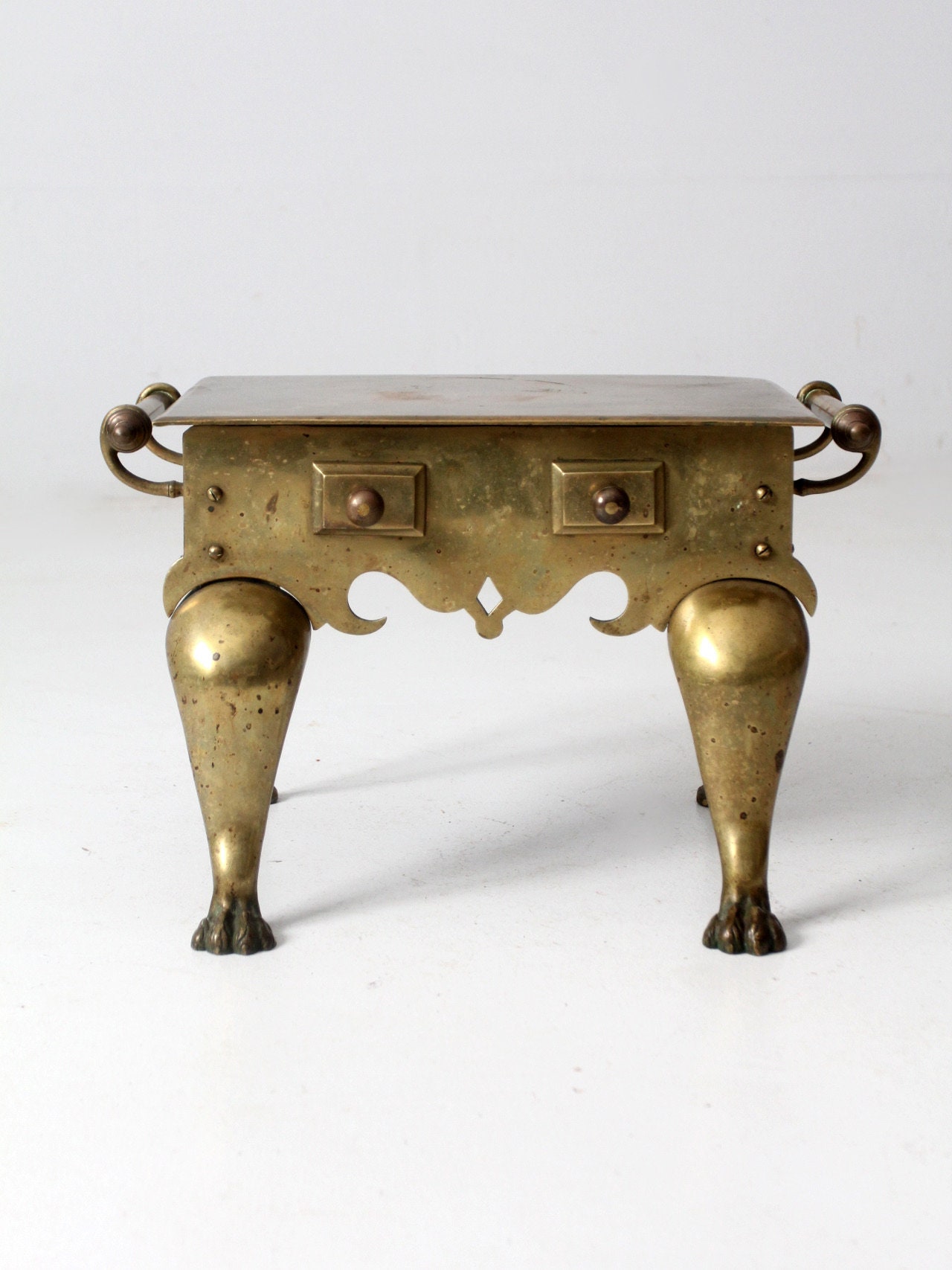The image is a color photograph showcasing a small, unique brass table with intricate detailing. Set against a white background with subtle shadows underneath, the brass table's surface stands out as the central focus. The table features ornate legs ending in lion's feet, and its aged, tarnished brass surface adds a touch of vintage charm. On either side, there are handles that rise up to the level of the tabletop, resembling grips. The table also includes two narrow drawers, each with a small knob, giving the table a functional yet decorative appearance. The combination of gold, brown, black, and gray hues enhance the antique feel of this distinctive piece, making it a striking object in what appears to be a product image likely photographed indoors.